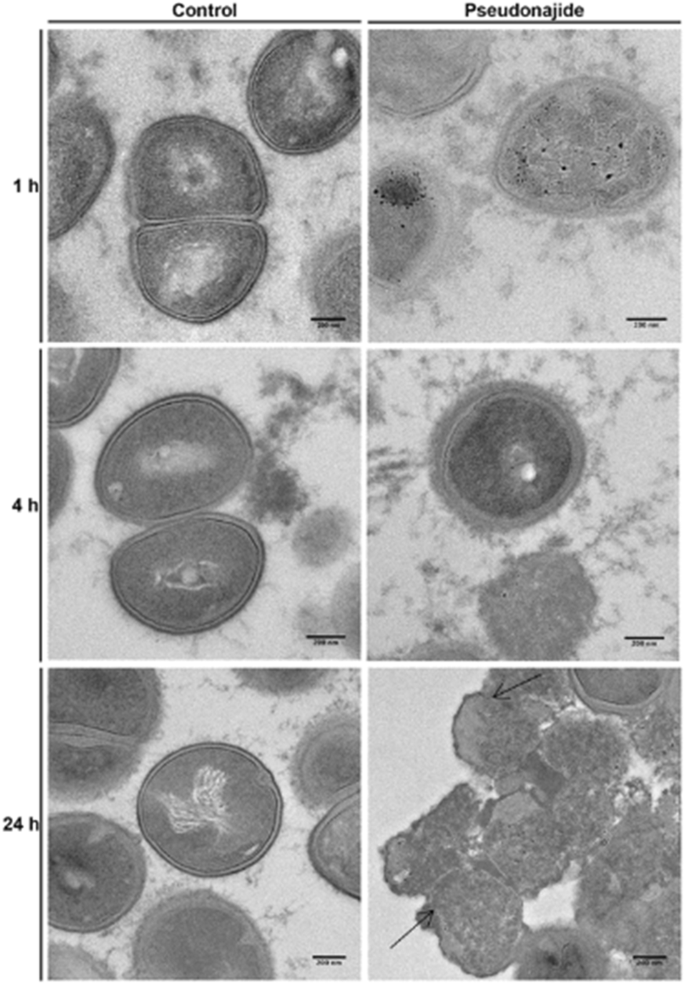This image displays six black-and-white photographs of cells under a microscope, organized into two columns and three rows. The left column is labeled "Control" at the top, while the right column is labeled "Pseudonagide." Each row correlates with different time points, marked as 1 hour (1H), 4 hours (4H), and 24 hours (24H) on the left side of the images. 

The top row features the initial cell configurations. The middle row shows cells in the process of division, with the control cells appearing to split while the pseudonagide-treated cells remain connected. By the bottom row, the control cells have divided into individual units, whereas the pseudonagide-treated cells form a large, dense mass. Each photograph also contains small, black, illegible text in the lower right corner.